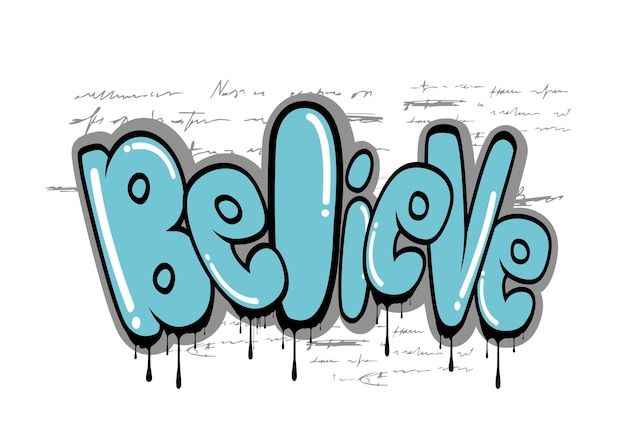This image is a piece of digital art featuring the word "BELIEVE" prominently in its center. The lettering is designed in blue, balloon-like, bubble letters, evocative of graffiti art. Each letter is bordered with a thick black outline that extends downward with a dripping effect, mimicking wet paint dripping in large globs. The word's design incorporates white accent lines around the edges, creating a reflection illusion. The letters also have a gray outline that adds a shadow effect, making the text appear three-dimensional. The interior of the letters, including the closed loops of the B's and E's, are filled in with the same shade of blue used for the primary lettering. The background resembles a piece of white paper covered in gray scribbles that match the gray of the letter outlines, giving a textured, hand-drawn appearance. This interplay between the detailed lettering and the scribbled backdrop suggests the image is inspired by graffiti and street art styles.